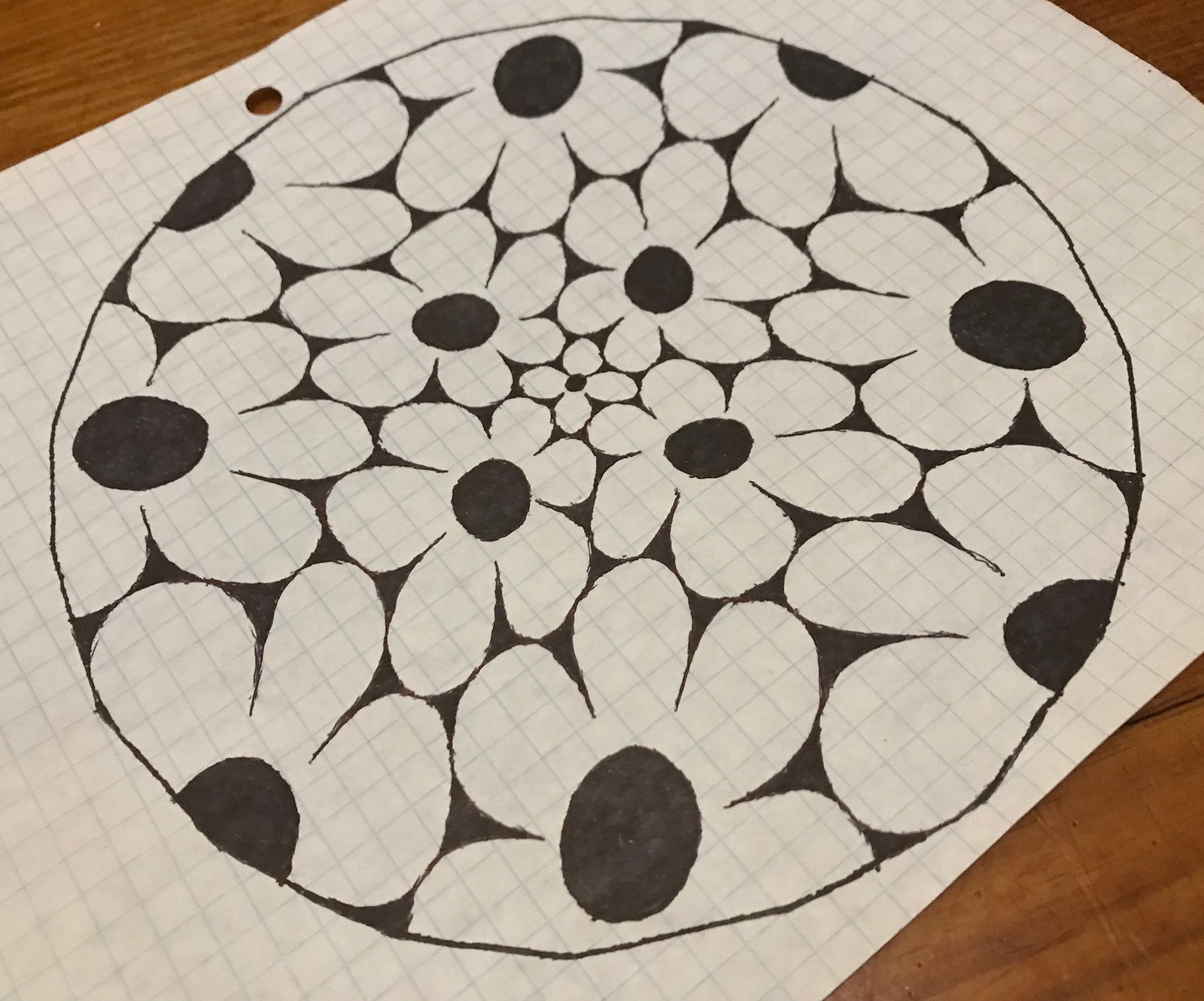The image features a detailed drawing of flowers on a single sheet of graph paper, appearing to be taken from a notebook due to the presence of a hole near the middle edge. The paper is placed on a dark brown wooden desk, with visible stains adding to the texture and character of the surface. The flowers dominate the paper, with the image slightly zoomed in. Each flower displays six petals with a black circle at the center, except for one smaller flower in the very middle, which uniquely has only four petals. The meticulous drawing contrasts with the subtle lattice of the graph paper, creating a pleasing and precise floral design.